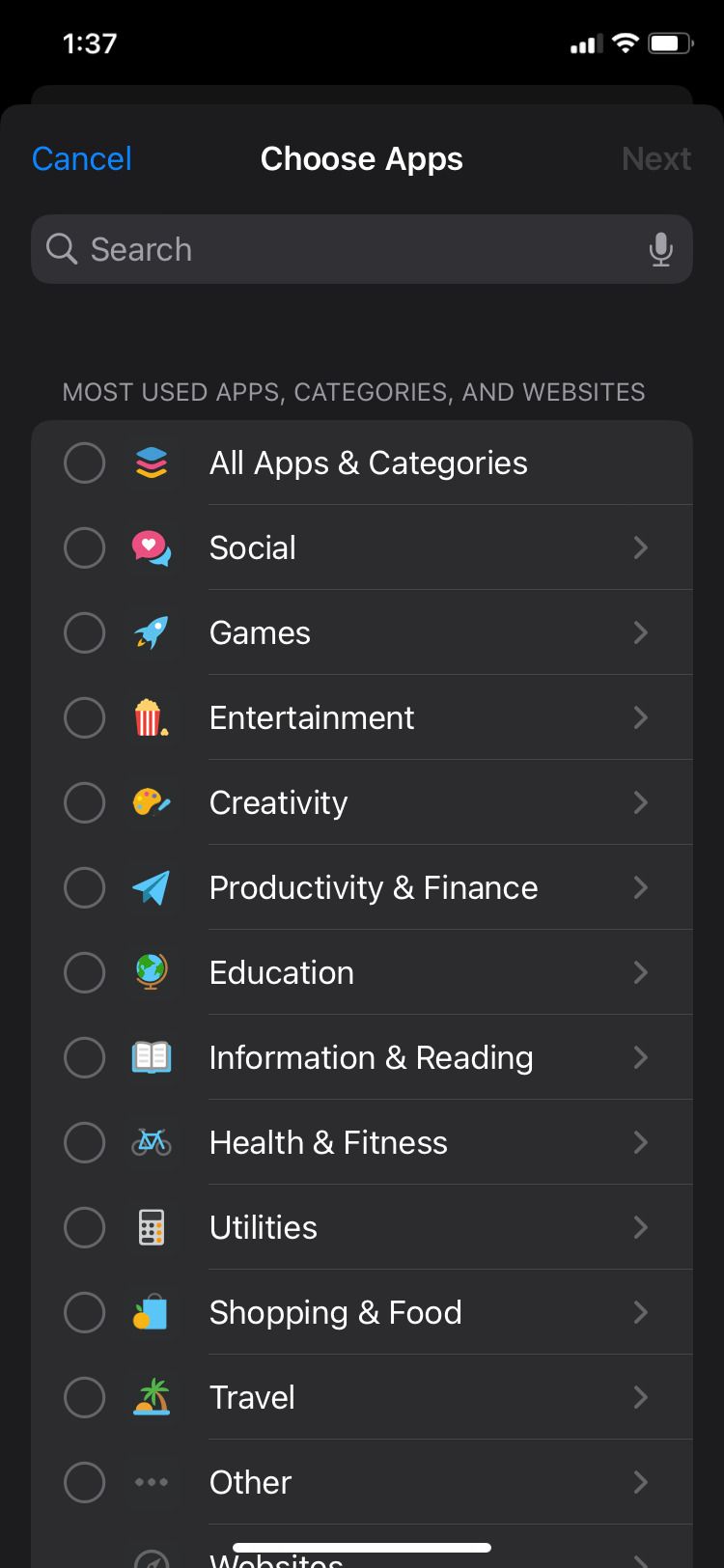**Screenshot Description: Mobile Phone Settings Screen**

The screenshot showcases a settings screen from a mobile phone interface, featuring a predominantly black background with white text. At the top left corner of the screen, the time is displayed as "1:37". On the top right corner, there are indicators for signal strength with 4 bars, WiFi with 3 bars, and a fully charged battery icon without numerical representation.

Beneath the status icons, on the left side, there is a "Cancel" option written in blue. Centrally placed, it reads "Choose apps". Just below this is a search bar for app navigation.

Further down, the screen categorizes options into "Most used apps, categories, and websites". Each category is followed by a list of apps, each indicated by an unticked round checkbox on the left and small white arrows.

The detailed categories and their icons are as follows:
- **All apps and categories:** 
- **Social:** No icon specified.
- **Games:** Illustrated by a rocket.
- **Entertainment:** Represented by what seems to be a cake or a present.
- **Creativity, Productivity, and Finance:** Displaying a paper plane.
- **Education:** Suggested by a globe icon.
- **Information and Reading:** Shown with a book icon.
- **Health and Fitness:** A small blue icon, specific shape not described.
- **Utilities:** Likely shown with a calculator.
- **Shopping and Food:** Indicated with an orange and a blue box.
- **Travel:** Depicted by a palm tree and some sea.
- **Other:** Marked with three dots.

At the bottom of the screen, there is a white line stretching across one-third of the screen centered horizontally. 

This detailed breakdown provides a comprehensive description of the various interface elements and organizational layout visible in the screenshot.